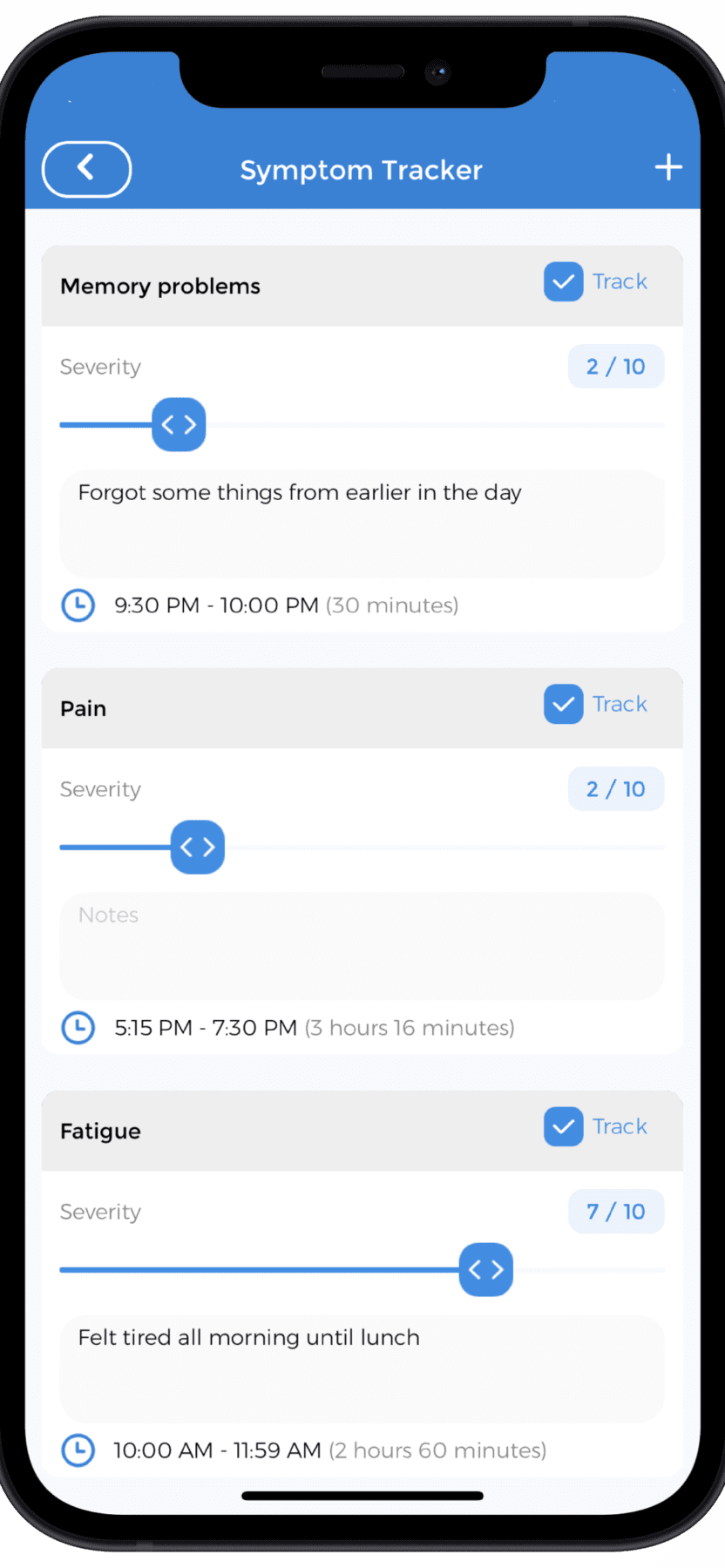The image displays a cell phone screen featuring a "Symptom Tracker" website. At the top of the screen, there is a prominent blue header with the text "Symptom Tracker" and a plus sign on the right side. Below this, "Memory Problems" is highlighted in a blue box with a white check mark. The severity is indicated as 2 out of 10, noting that the user forgot some things from earlier in the day. The timestamp for this entry is from 9:30 to 10:00 PM, totaling 30 minutes.

Further down, there is another blue box with a white check mark labeled "Pain." The severity listed here is 2 out of 10. Below this entry, a section labeled "Fatigue" is marked with a blue box and a white check mark, showing a severity of 7 out of 10 with the note "Felt tired all morning and lunch." 

A small blue circle icon displays the time between 10:00 AM and 11:59 AM, indicating a duration of 2 hours (120 minutes). The overall screen is bordered by a black liner, characteristic of a phone, with the current time displayed at 10:00 AM in the upper right-hand corner. A counterclockwise arrow icon is also present at the top right, symbolizing refresh or reset.